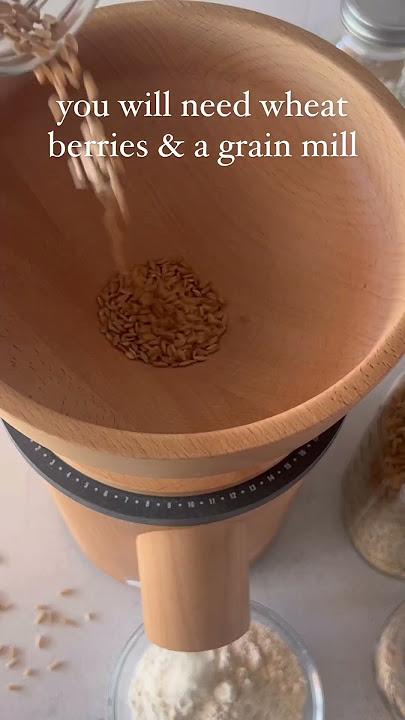In this detailed image from a cooking series, a tall wooden grain mill stands on a white counter. The grain mill features a round chute from which freshly ground white flour is dispensed into a clear glass bowl beneath it. Scattered grains are visible on the counter beside the bowl. Around the top of the grain mill, a black ring with various numbers indicates the settings for the fineness of the grind. At the top of the mill, there is a wooden bowl with a hole where someone is pouring wheat berries from a clear glass container. In the background, there are three or four clear glass mason jars with different grains, each sealed with a silver lid. White text at the top of the image reads, "You will need wheat berries and a grain mill."